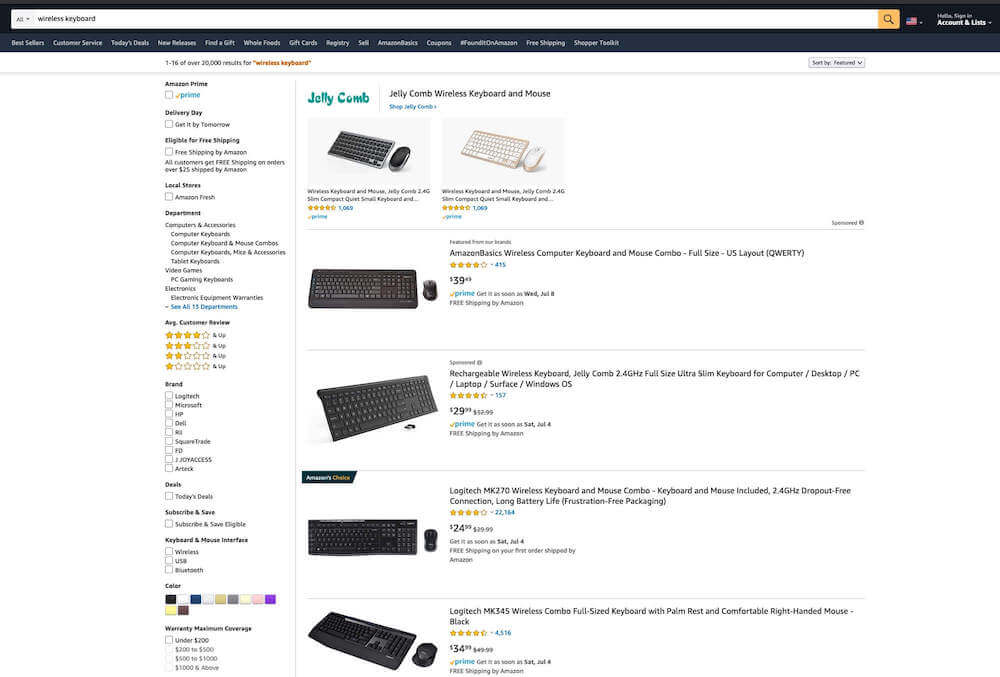The image depicts a website resembling the layout of Amazon's online store. Prominently featured is a list of keyboards. The first item displayed is the "Jelly Comb Wireless Keyboard and Mouse." Next in line is the "Amazon Basics Wireless Computer Keyboard and Mouse Combo (Full Set, US Layout)," noted for having slightly smaller writing on its description, including a few letters in parentheses. This combo is priced between $39.99 and $65. Another item listed is a "Rechargeable Wireless Keyboard" from Jelly Comb, with a noted 2.4 GHz wireless connectivity.